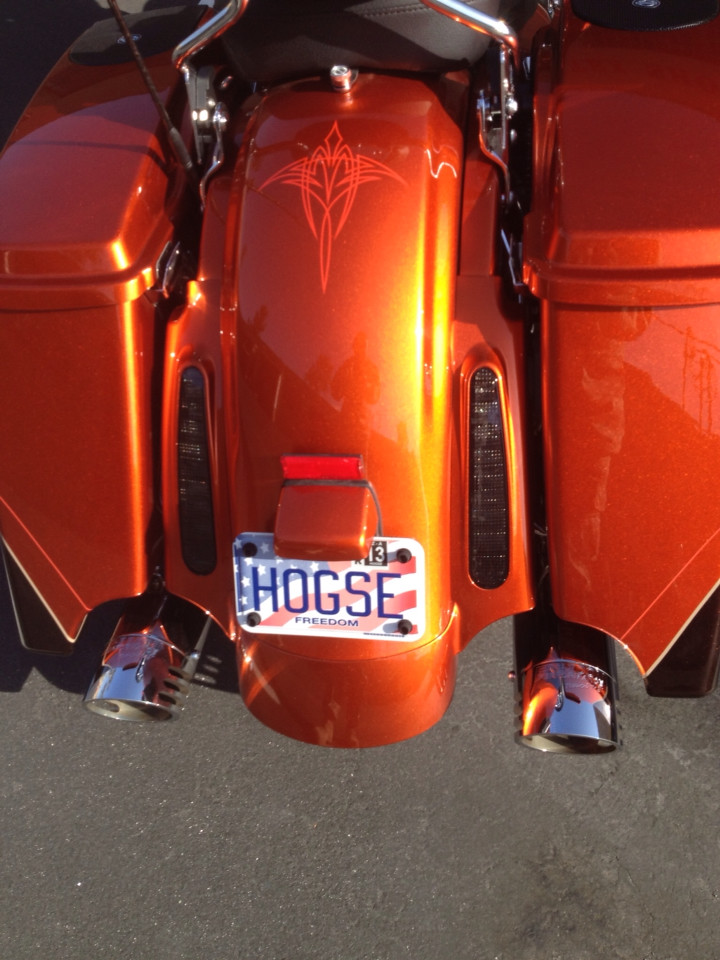This photograph captures the striking rear end of a bright reddish-orange motorcycle, gleaming under the bright sun and parked on dark gray pavement. Dominating the center, the license plate reads "H-O-G-S-E," with an American flag backdrop and the word "Freedom" emblazoned underneath—a poignant emblem of liberty. The plate's top also features the number 13, potentially indicating the year 2013. Flanking either side of the plate are two shiny silver exhaust pipes, and above them, two rearview lights. The motorcycle's rear showcases two horizontal metal saddlebags, suggesting ample storage. Despite some uncertainty about whether it's a standard motorcycle or a trike, it's clear that the vehicle's new, meticulously polished appearance and its intricate chrome hardware leave a lasting impression. The fender, along with a visible black bottom strip and a metallic bar hinting at a passenger seat's support, add to the detailed layout captured in this crisp image. The entire composition is neatly framed, focusing on the license plate and exhausts while cropping just above the saddlebags.